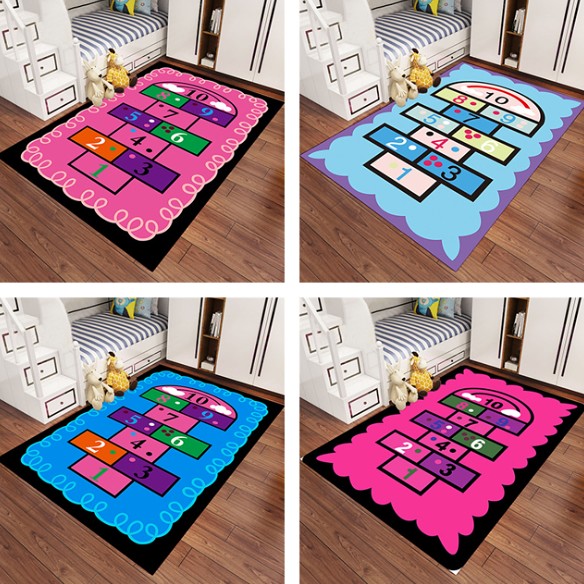In this image, we see four kid bedrooms, each featuring a neatly arranged bed. The bed has white and striped bedding with a blue pillow. Next to it, on the floor, there's a yellow and white stuffed animal. The bed is part of a bunk setup with steps on the left side that double as drawers. These stairs are white, matching the rail attached to them. 

Each room showcases a different hopscotch-themed rug positioned on a dark brown wooden floor. All the hopscotch rugs have the numbers 1 through 10 arranged from bottom to top, with alternating single and double rectangles. The top left corner of the image features a rug with a pink interior and a black border. The top right corner showcases a rug with a teal interior and a purple border. The bottom left has a rug with a blue interior and a black border, while the bottom right rug has a pink interior and a black border. The borders of these rugs vary, including decorative elements like curls or string-like designs.

Additionally, in the top right corner of the room, there's a closet providing extra storage space. This image beautifully captures the harmony between functionality and playful design in these children's rooms.